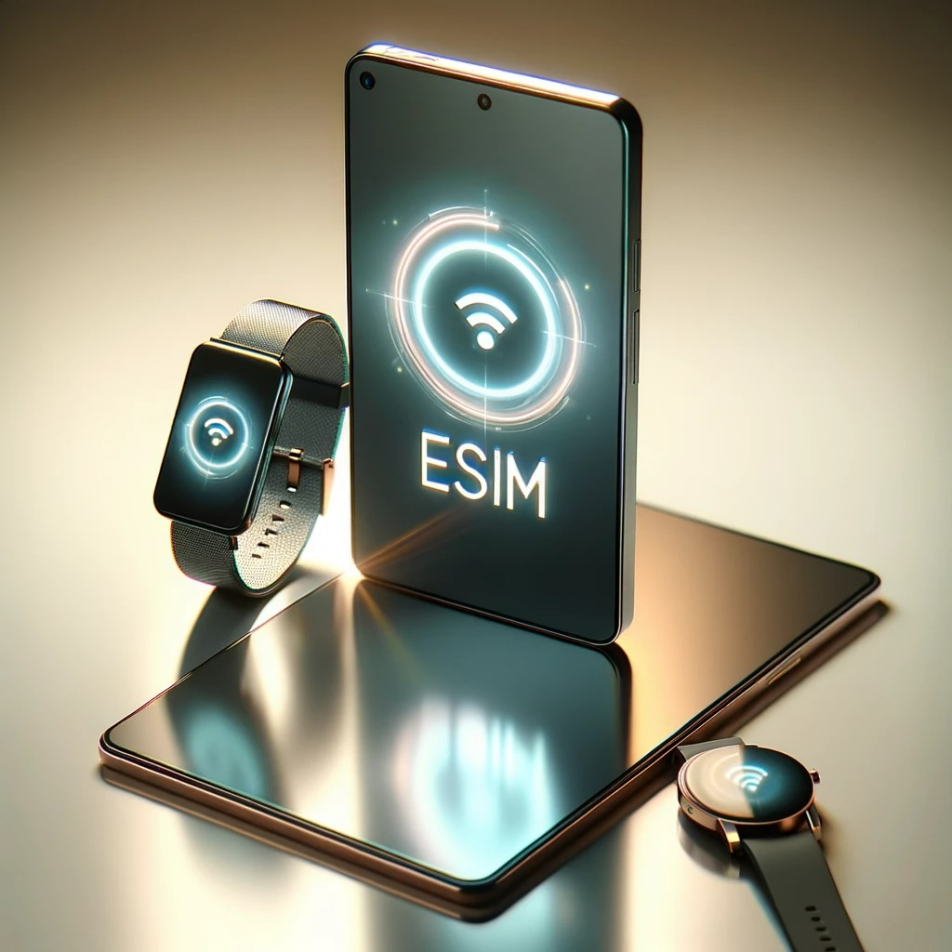The advertisement showcases an intricately rendered 3D image of a sleek, black, and dark silver smartphone branded with the logo "ESIM". The phone, prominently displaying signal strength bars and vibrant, fiery graphics around the emblem, is standing upright on a tablet-like device. Flanking the smartphone are two smartwatches that similarly feature the ESIM logo and signal graphic on their screens. The watch to the left of the phone has a rectangular shape while the one on the right is round. This composition is set against a minimalistic, detail-free background to keep the focus on the devices, emphasizing the cohesive and branded aesthetic of the ESIM technology lineup.